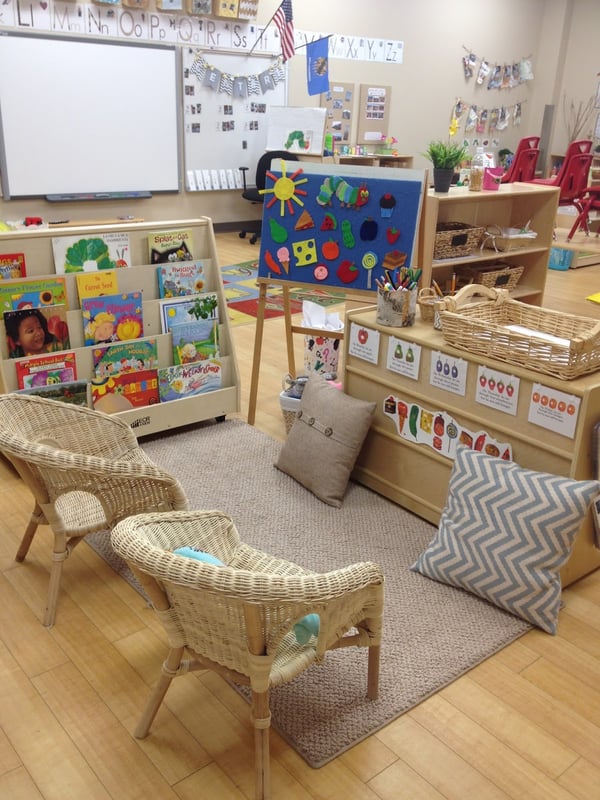The image depicts the interior of a bright and inviting kindergarten or pre-K classroom. The walls are painted white, and a whiteboard occupies a prominent place, adorned with the alphabet above it. An American flag and a blue state flag also hang nearby. Words can be seen on the board. Red chairs are stacked in the background, and there's a tan shelving unit on which a plant is placed, along with baskets tucked into the shelves. Near the front of the room, a cozy reading area features a tan bookshelf filled with children’s books, two tan wicker seats, and a brown rug with two throw pillows atop it.

An easel stands in the center, displaying an array of colorful objects, including a depiction of the 'Very Hungry Caterpillar,' along with drawings of the sun, cheese, ice cream, and sausages, possibly part of a lesson or story display. To one side, there's a setup resembling a cashier's counter, likely intended for imaginative play. This classroom setup, complete with woven seats and educational signage on cabinets, fosters an engaging and nurturing environment for young learners.